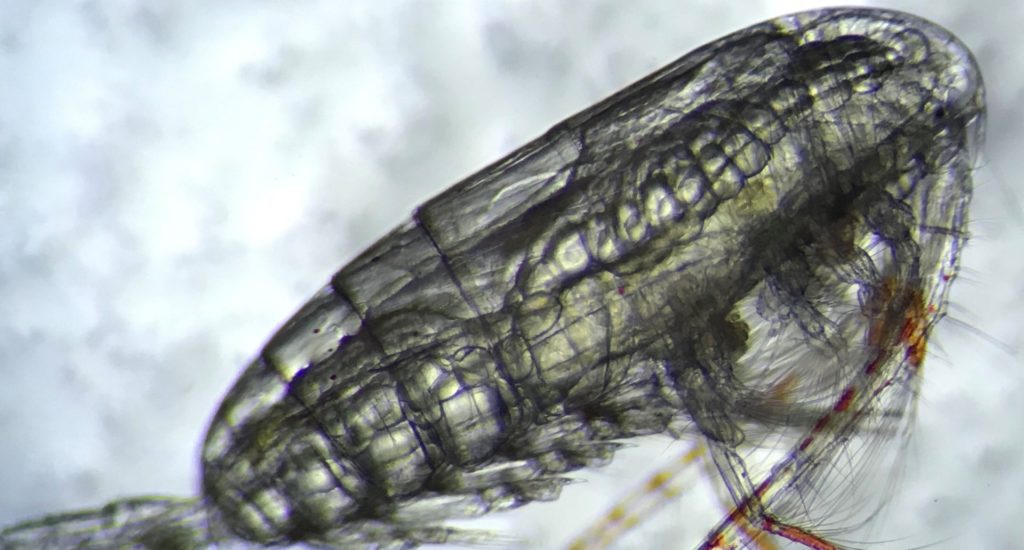This close-up, potentially microscopic image showcases a transparent bug, presenting an almost x-ray-like view. The creature, possibly a dust mite or similar insect, reveals its inner structure through varying translucent shades of gray, white, and a touch of tan and brown along the body and legs. The bug's pill-shaped form lacks distinct segmentation, yet a spine-like feature runs from head to midline. Its appearance combines elements reminiscent of a snake's ridged head and a fly's legs, some parts adorned with possibly hairy or stringy appendages near the mouth, highlighted subtly in orange. The blurred, off-white to gray background further accentuates the detailed internal greenish bead-like structures of the bug, offering a glimpse into its intricate anatomy.